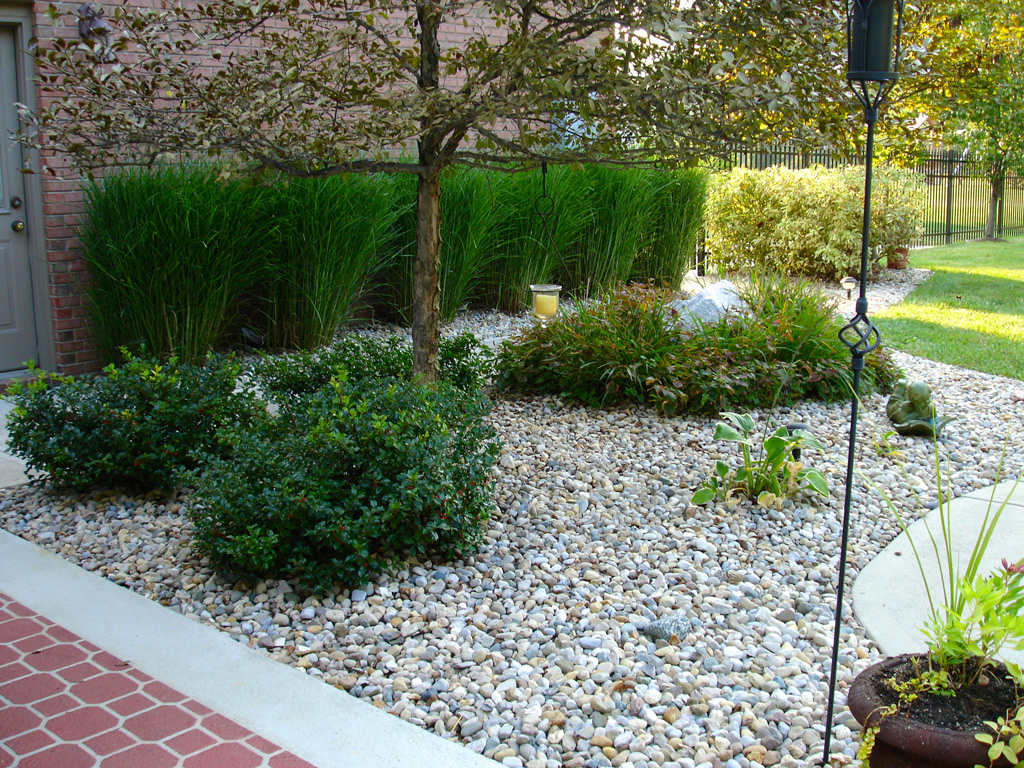A vibrant outdoor photograph captures a sunlit landscape featuring a diverse array of green foliage. Prominently positioned in the center, a spacious tree with sparse leaves stands amidst a gravel bed, receiving ample sunlight due to its significant size. Surrounding this tree are a collection of smaller bushes, varying in shades of green, from deep hues to lighter tones. These plants rest on a reddish-brown brick ground that extends into a path bordered by concrete on the bottom left. To the right, tall grasses, some possibly taller than a human, are seen behind a black fence, leading into a field. Adjacent to this verdant display, a red brick building rises, boasting additional bricks along its side for continuity. This structure features a gray wooden door equipped with a brass doorknob and deadlock on its left side, while several medium to large green bushes buffer the building’s facade. The image harmoniously blends natural and architectural elements, creating a richly detailed and picturesque scene.